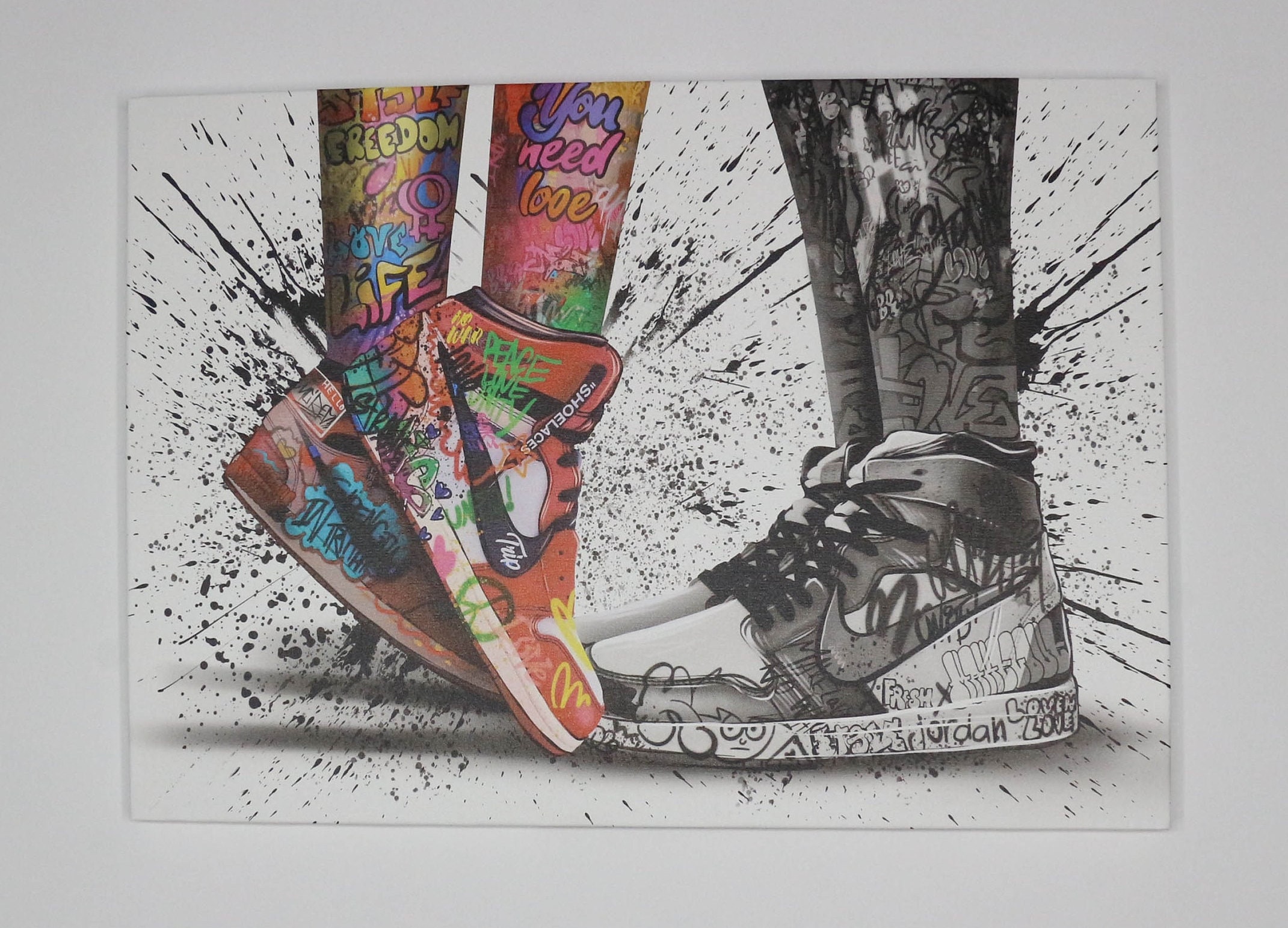This image portrays a vibrant piece of artwork, possibly an acrylic painting or a printed work displayed on a white wall, bordered by a gray frame. The scene focuses on two pairs of legs and feet, depicted from mid-shin down, positioned against a white background splattered with black ink. The left pair of feet, likely female, is adorned in brightly colored red Nike sneakers with a distinctive black Nike swoosh. These sneakers are embellished with a peace symbol and various colored writings, including affirmations like "You Need Love," "Freedom," "Love," and "Life." The legs are similarly decorated with bold and colorful designs and graffiti-like text, displaying shades of yellow, red, pink, and orange. Notably, this left figure is partially standing on tiptoes, emphasizing the dynamic posture.

Contrastingly, the right pair of feet and legs, likely male, are rendered in black, white, and gray tones. The sneakers, resembling Nike Air Jordans, feature a mix of dark gray with white accents, including the tip and sole. These shoes and the legs also exhibit graffiti-style drawings, though in monochromatic hues. The feet on the right are flat on the ground, providing a stark, grounded contrast to the colorful and lifted posture of the left pair. The entire composition juxtaposes lively and muted elements, connected by the recurring theme of street art and graffiti, creating a striking and balanced visual narrative.